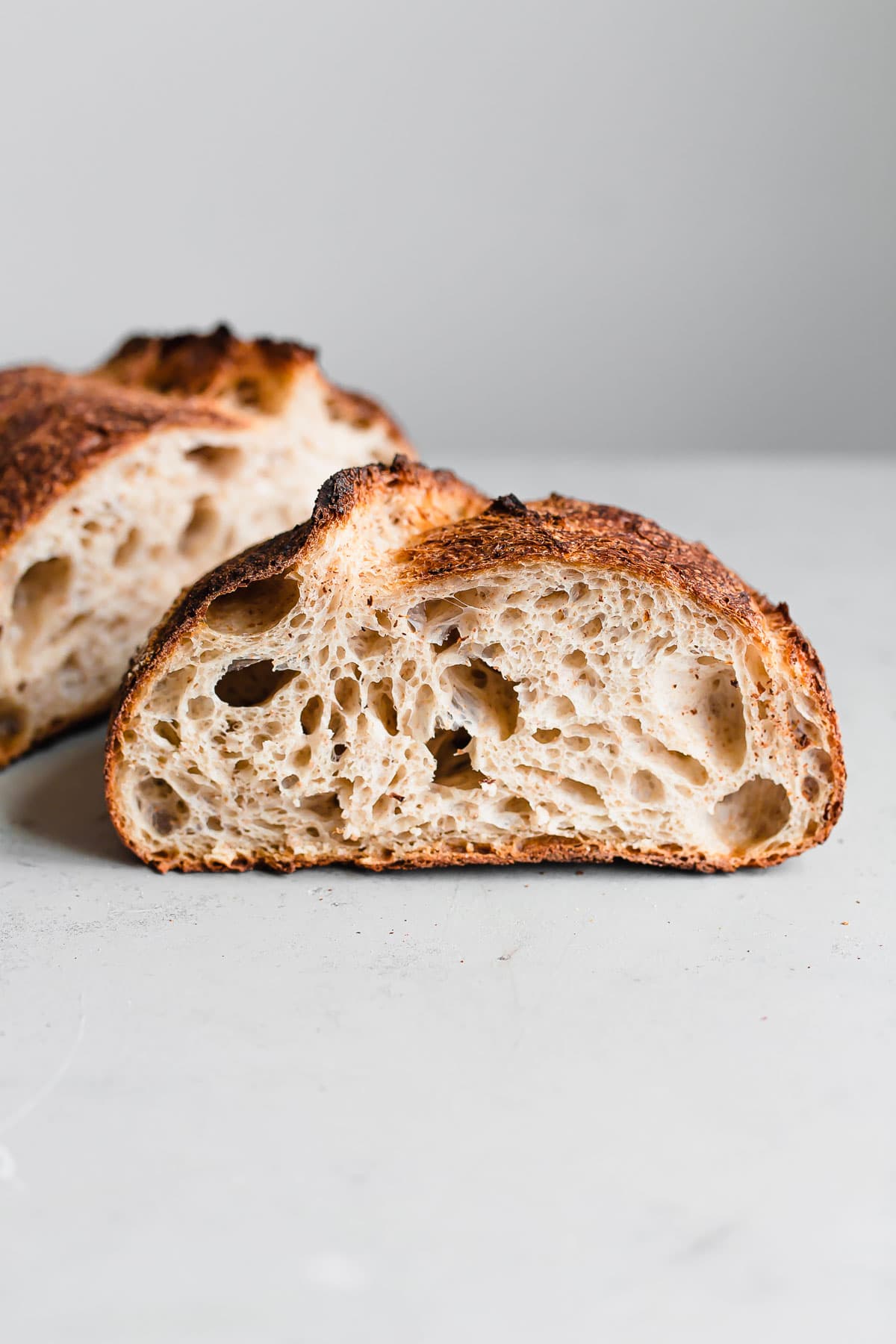The photograph showcases a small, rustic loaf of bread that has been sliced into two halves, placed on a flat gray surface with a matching gray background. The primary focus is on the foreground slice, centered and sharply in focus. This slice, characterized by a dark brown, crisp crust with slightly burnt edges, contrasts with its soft, golden creamy interior, marked by large air bubbles and pockets indicative of thorough fermentation. The bottom of this slice is flat, while the top is rounded with a small 'ear' where the crust has pulled away during baking. The second half sits behind the first, at a 45-degree angle, slanting from the bottom left to the top right of the photograph. Despite its rustic appearance, the bread's texture and presentation evoke a sense of deliciousness, hinting that it could pair wonderfully with cheese and wine. The overall simplicity of the scene—two slices of delectable bread against a neutral background—draws the viewer's attention to the intricate details of the loaf's craftsmanship.